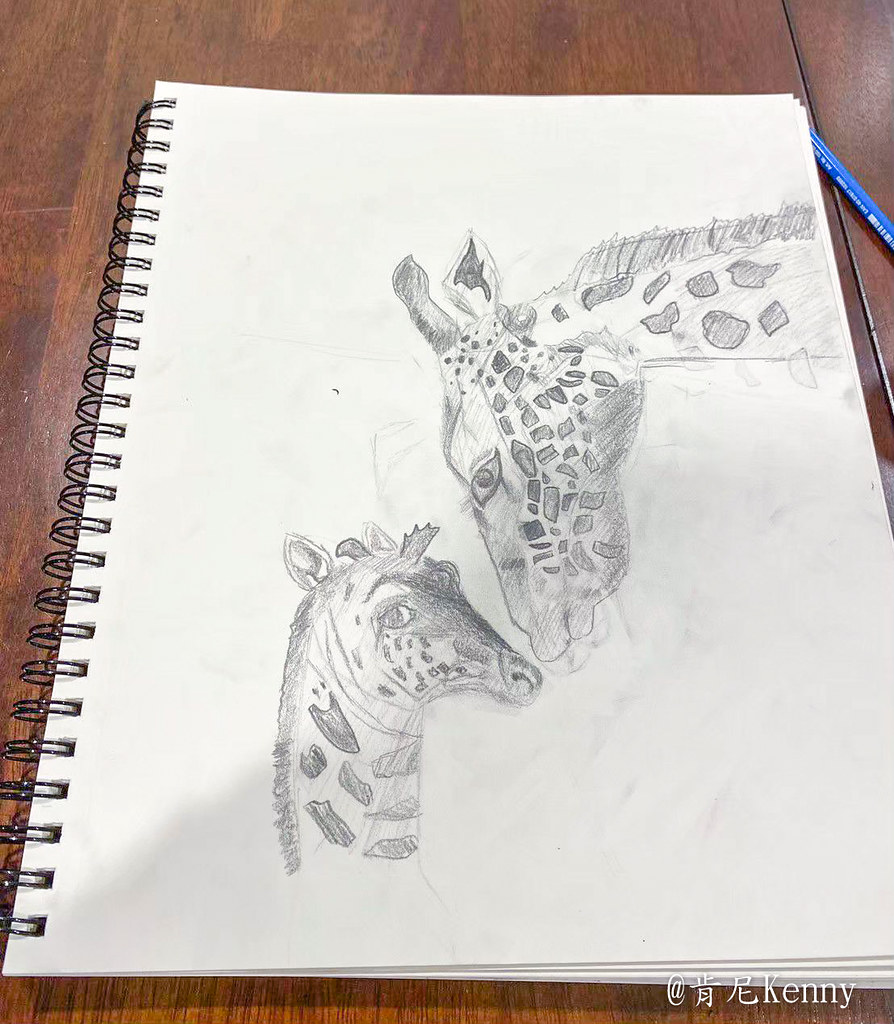This beautifully crafted pencil drawing features an endearing scene of a baby giraffe and its mother. The tender moment captures the two giraffes as they lean towards one another, almost touching heads, conveying a sense of affection and connection between them. The baby giraffe's gaze appears to be directed towards the viewer, adding an engaging and intimate touch to the composition. Meanwhile, the mother giraffe is focused on her offspring, exuding a nurturing presence.

In the bottom right corner of the drawing, there are two Chinese symbols, followed by the signature "Kenny" in capital letters, indicating the artist's identity. While the artwork demonstrates a commendable level of skill, especially in the depiction of the giraffes' forms and expressions, there is room for improvement in the shading and detailing of their fur. Despite these areas for enhancement, the drawing remains a charming and heartfelt portrayal of a mother-child bond in the animal kingdom.